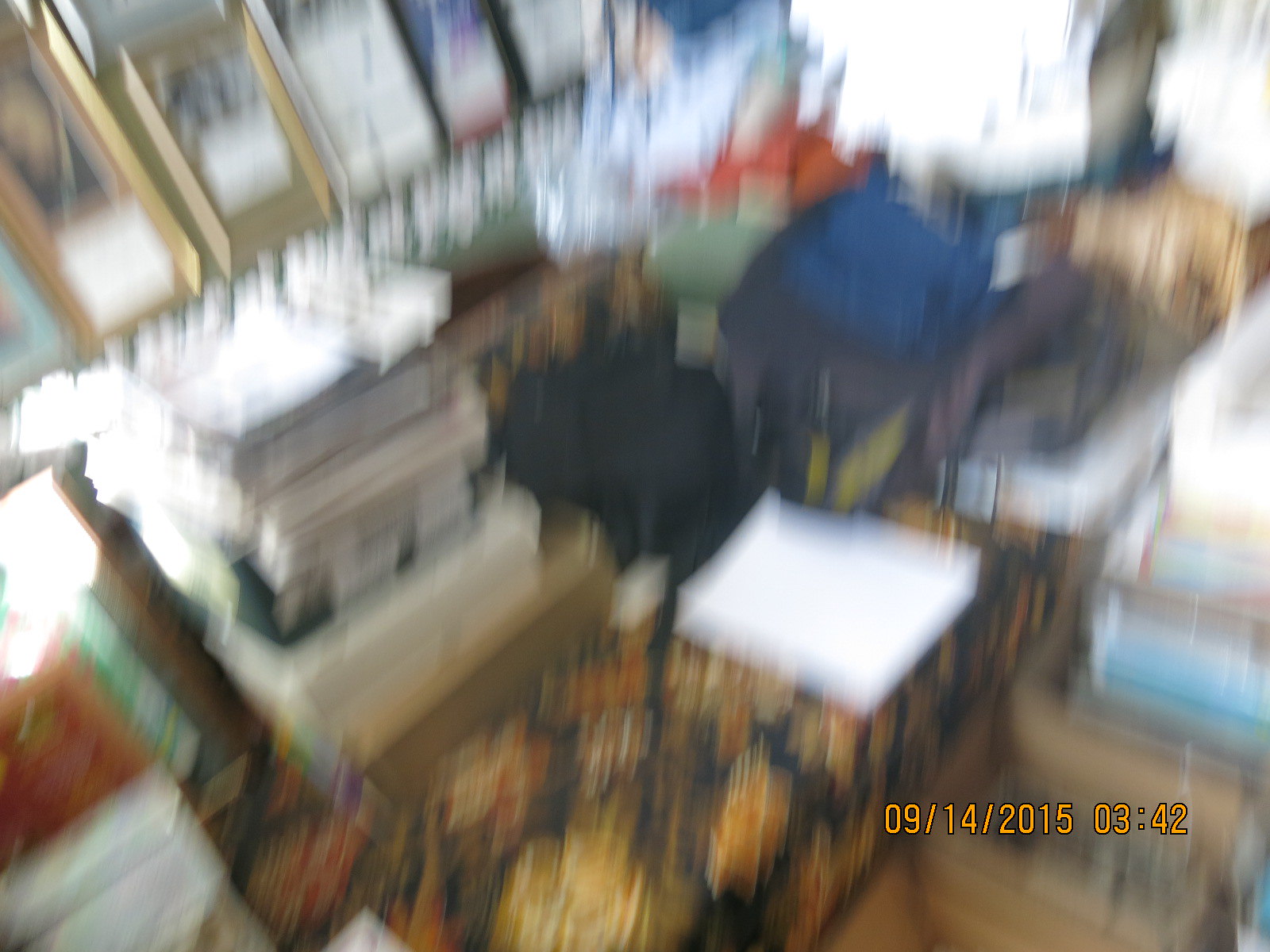This blurry security camera footage, dated September 14, 2015, at 03:42, captures what appears to be the interior of a store. The timestamp in the bottom right-hand corner is prominently displayed in orange text with black outlining. Despite the image's low quality, several details emerge: The background features a dark green wall adorned with various rectangular picture frames in colors like gray, white, and even some showing purple hues. Below these frames, a long table or possibly a bench with a black floral-patterned cloth can be seen. The cloth has noticeable orange and yellow-brown splotches. On this surface, there are piles of papers and books, possibly including a blue bag and several white sheets of paper. To the right, a stack of brown boxes and clear bins is visible, hinting at a cluttered yet organized space.